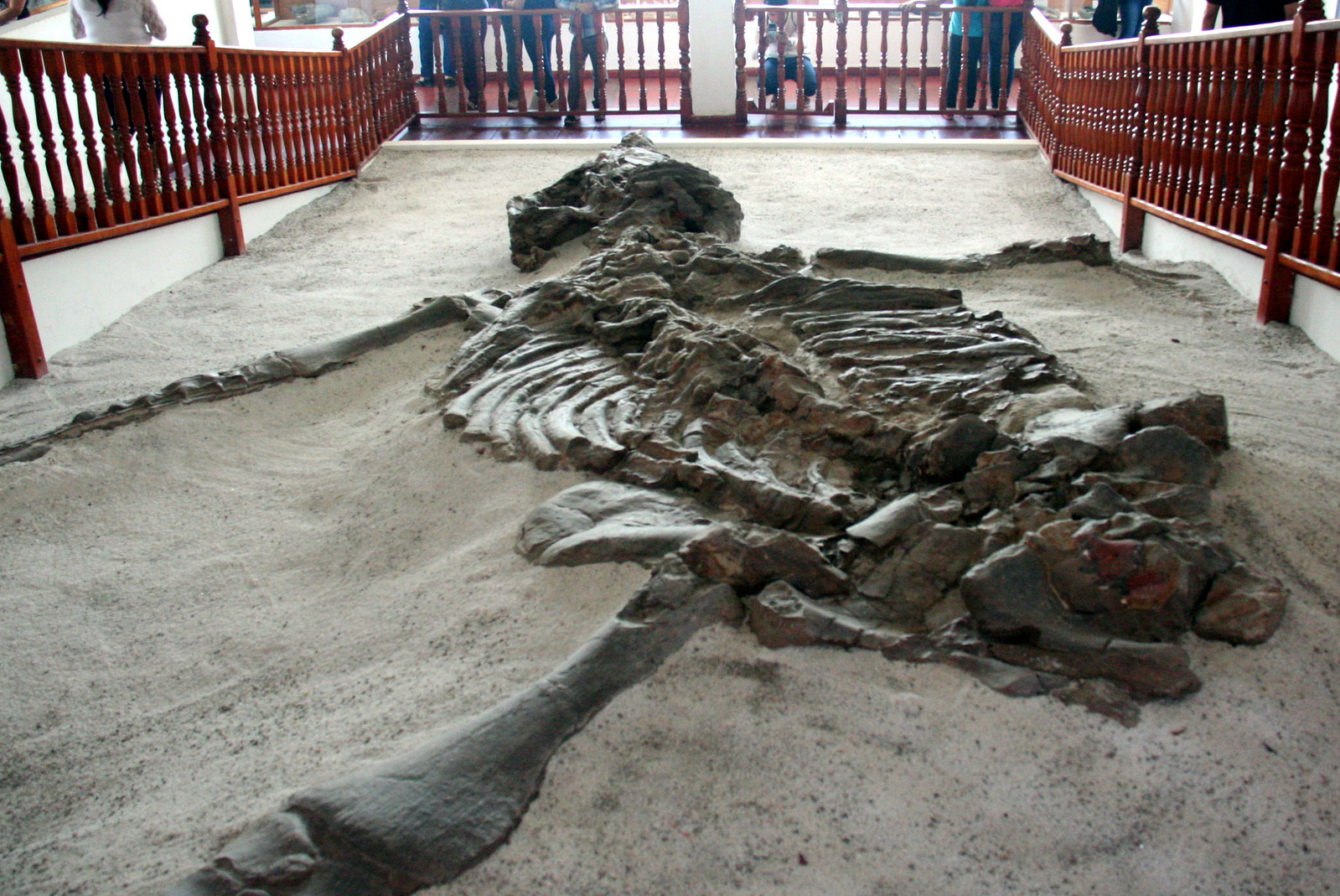In this image, a well-preserved skeleton, likely of a turtle or an aquatic creature with flipper-like limbs, is meticulously displayed in a clear bed of sand. The exhibit is surrounded by a low red fence, approximately two to three feet tall, designed to prevent visitors from accessing the display area. The scene is framed by a back wall at the top of the image, where the legs and torsos of some onlookers are visible, providing a sense of scale and perspective. The skeleton appears to be almost complete, and is carefully laid out to showcase its structure, creating an informative and intriguing presentation for the viewers gathered around the fence.